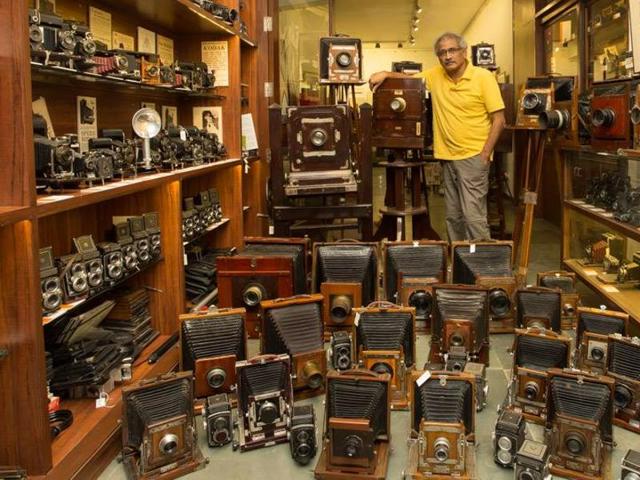In the heart of a vintage camera museum, an older gentleman stands proudly amidst a vast collection of antique photography equipment. Dressed in a yellow collared shirt and grey pants, with glasses perched on his nose and white hair framing his face, he positions himself beside an impressively large, old-timey camera, resting his arm affectionately on it. The room around him is a treasure trove for any photography enthusiast, filled with cameras from the 1800s to the 1920s. Shelves upon shelves, some glass-encased, display an array of cameras and camera flashes. There are double lens cameras on one side, while the floor is strewn with even more vintage pieces. Display lights from the ceiling illuminate this expansive assemblage, highlighting the historical significance of these early photographic devices. This scene, possibly his store or a cherished collection space, captures the essence of a bygone era in photography.